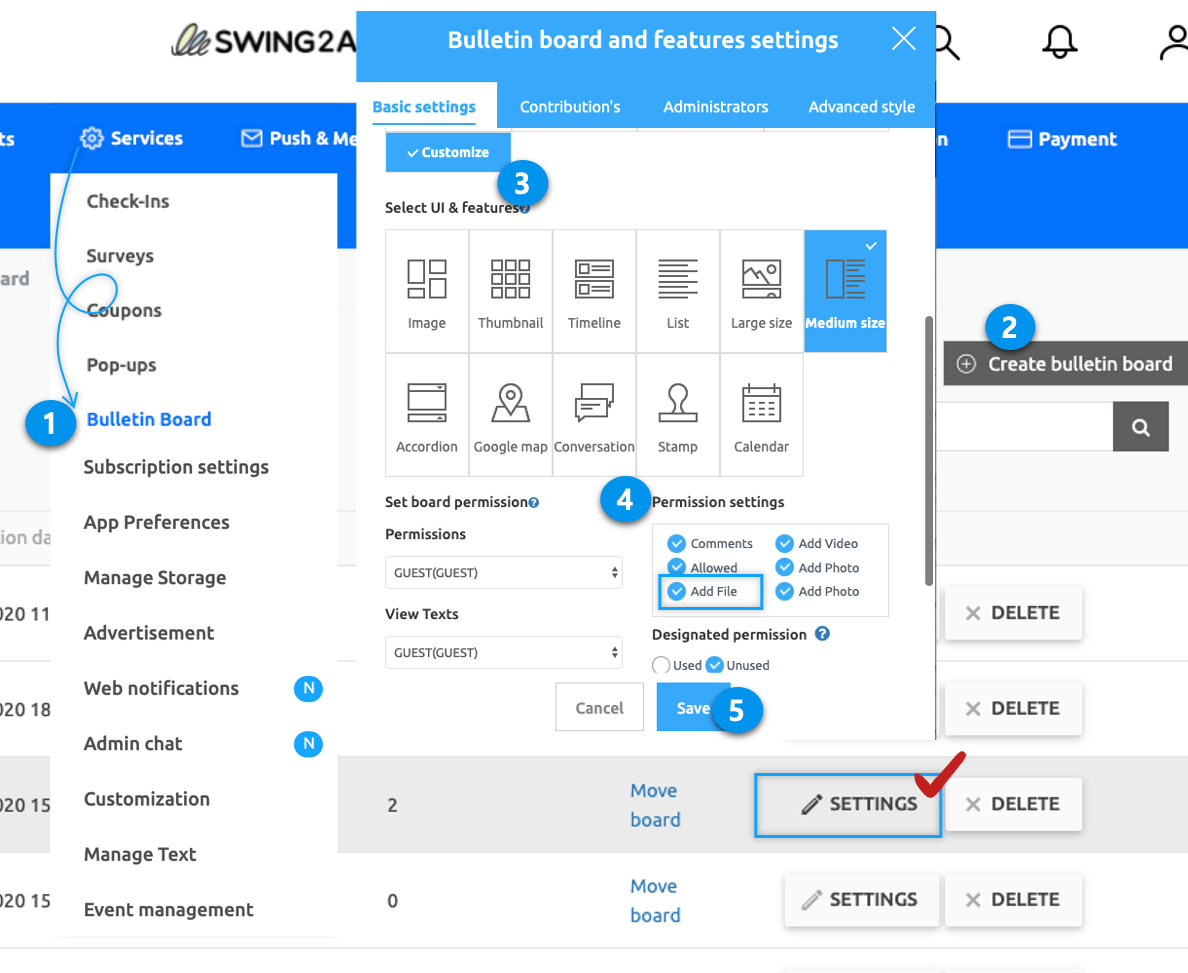This intricate image showcases an overlay of multiple cutouts from a website, each meticulously detailed to create a layered visual effect. Dominating the scene, the base layer reveals a white header adorned with notable elements. On the top left, bold black text reads "SWING2A" in all caps, accompanied by a charming cartoon-style spring icon. This header, however, is partially obscured by an overlapping popup window.

To the right of the concealed text, a series of medium gray icons punctuate the white header. These include a search/magnifying glass icon, followed by some spacing, a bell icon, and finally, a person outline icon, each spaced evenly apart.

Beneath the white header, a striking blue bar runs across the screen. On its top left, a white cog icon sits next to the word "SERVICES" in crisp, white lettering. Further right, spaced out in a minimalistic fashion, appears a white envelope icon with the phrases "PUSH" and "ME" beside it. The rest of the text is eclipsed by the popup, except for a visible letter "N," a white credit card icon, and the word "PAYMENT" on the far right.

The center of attention is the popup window, which features a lighter blue header with prominent white text reading "BULLETIN BOARD AND FEATURES SETTING." Just below, four tabs are arranged horizontally, the first of which is selected and highlighted with a white background and blue text, stating "BASIC SETTINGS." Adjacent to it, the other tabs, "CONTRIBUTIONS" (notably with an apostrophe between the N and S), "ADMINISTRATORS," and "ADVANCED STYLE" share the blue header’s background color and feature white text.

The body of the popup window itself possesses a clean white background, populated with dark gray icons and text, organized to convey information seamlessly to the viewer.

In sum, this detailed image encapsulates the organized chaos of a website's interface, layered intelligently to focus attention on pivotal elements and navigation icons.